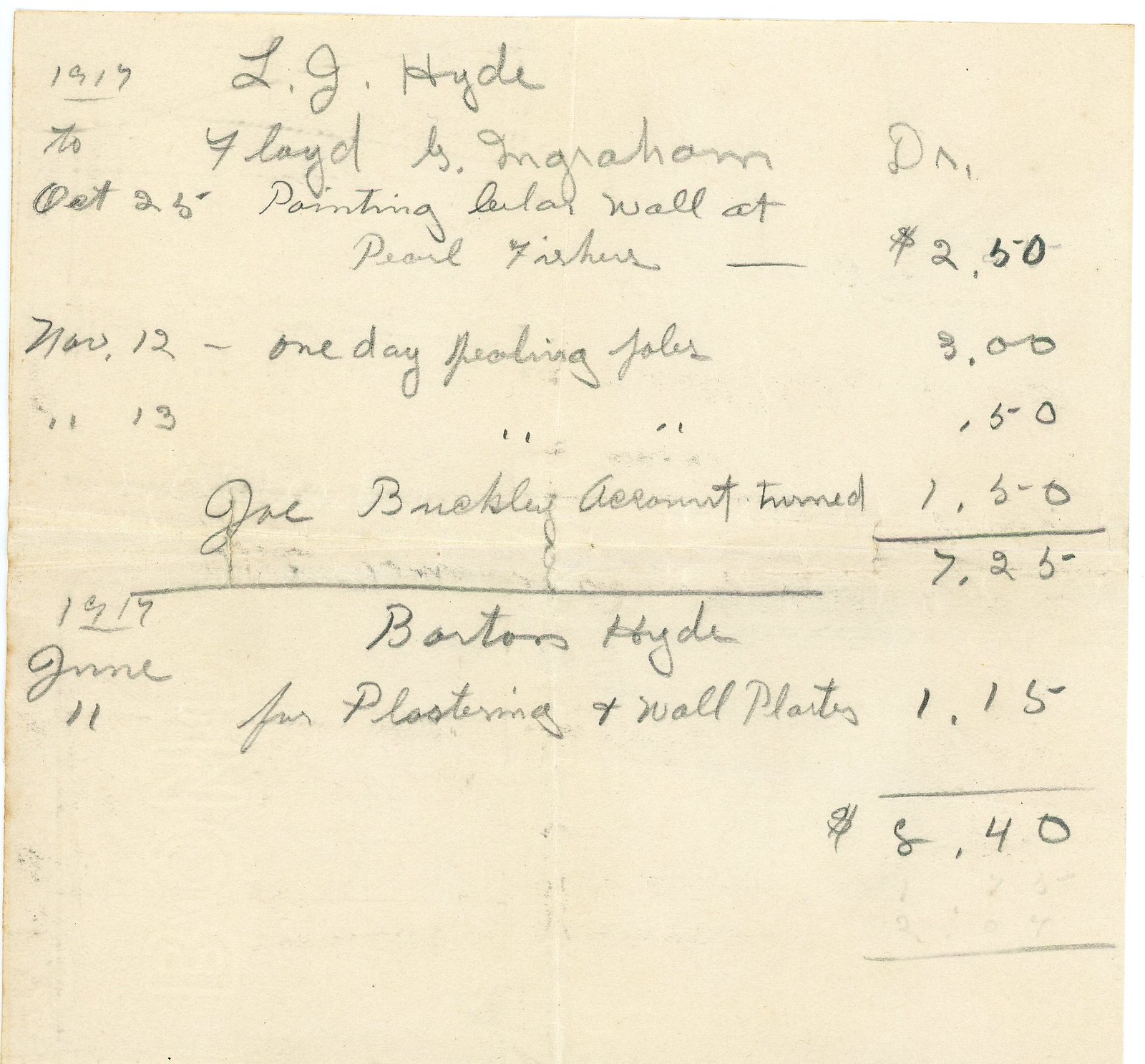The image features an off-white, dingy piece of paper covered in gray pencil markings and cursive handwriting. The paper appears to contain various dates, names, and monetary amounts, indicative of a messy, partially erased accounting record. At the top left, the date "October 25th, 1917" is visible, followed by another date, "November 12th," just below it, and "June 11th, 1907" further down. Along the left side, names like "LG Hyde" and "Barton Hyde" are mentioned next to notes such as "plastering of wall parts or plants" and other work details that are less legible. The right side of the paper lists monetary amounts: $2.50, $3.00, $0.50, and $1.50, adding up to $7.25, with an additional $1.15 noted below, totaling $8.40 in a box at the bottom right. Despite the smudges and the difficult-to-read handwriting, the paper seems to be an old ledger or financial record, detailing various expenses and tasks from the early 20th century.